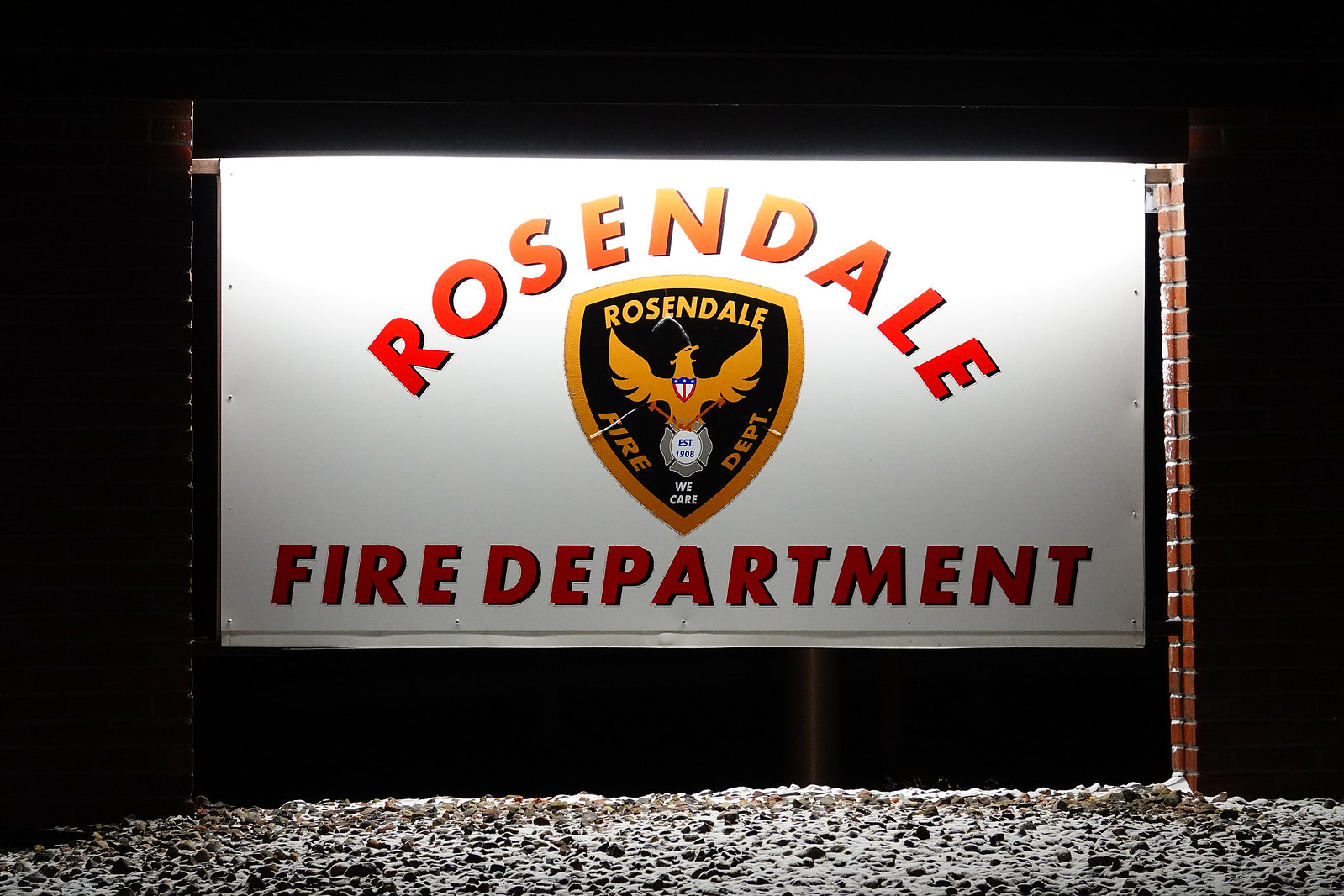A photograph of an outdoor sign for the Rosendale Fire Department, securely mounted on two brownish-red posts set into a gravel or rocky base, which suggests a dark or nighttime setting. The sign is horizontally rectangular and made of a vinyl material with a white background. "Rosendale" is prominently displayed at the top in large, capital letters that transition in color from red at the edges, through orange, to yellow at the center. This text is arched slightly to form a semi-circle. Below this text is a centrally-located gilded gold emblem with a black background, featuring a yellow eagle with spread wings. The eagle bears a crest resembling the American flag on its chest and stands above a smaller white and black emblem. Alongside the larger emblem's border, the word "FIRE" is inscribed on the left, and "DEPT." on the right. At the emblem's base, in white text, it reads "We Care." At the bottom of the sign, in red letters with a black shadow, the words "FIRE DEPARTMENT" are displayed prominently. The sign overall measures approximately four feet wide by three feet high, with about a foot of space between the ground and the sign's lower edge.